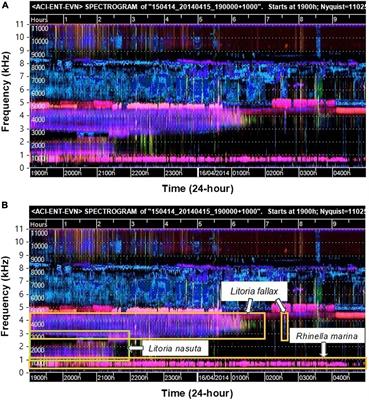The image depicts two horizontally-aligned charts, one on top of the other, each slightly longer than they are tall, and set against a plain white background. The overall dimensions of the image are roughly three inches high and two inches wide. Each chart features a black header and footer with white text; the top chart is labeled "ACIONEVN spectrogram of 15041420140415. 190,000 plus 1,000 starts at 1900H, Nyquist 1102," and the bottom chart bears the same title. Both charts span a 24-hour period, with the x-axis representing time in hourly increments (1900H, 2000H, 2100H, etc.) and the y-axis labeled as "frequency, kilohertz."

Chart A and Chart B are distinctly marked, with A on top and B at the bottom. Both charts showcase a spectrum of colors, including strands and bars in hues of pink, purple, blue, and white. Chart B distinctly features outlined yellow sections, with white rectangles pointing to areas of interest, labeled "Litoria Nasuta," "Litoria Falix," and "Rainella Marina." The charts are visually detailed, with intricate colored lines and sections providing a visually rich representation of the frequency data over time.